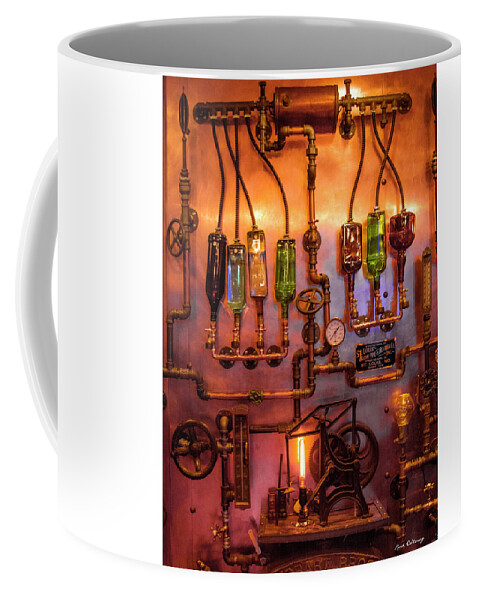This image depicts a white mug with a detailed, intriguing illustration on its surface. The image seems to represent a complex and industrial scene, reminiscent of a distillery or a mechanical control room. The centerpiece of the illustration is an intricate system of interconnected golden pipes, adorned with various gauges, dials, and control wheels that resemble steering mechanisms used to regulate flow and pressure. Below the pipes lies a workbench area equipped with a torch lantern and assorted tools, enhancing the industrial vibe. Prominently featured within the pipe system are multiple vials filled with different colored liquids, connected by wires to a device positioned at the top. These vials appear to be similar to liquor bottles such as wine or scotch, adding a unique and colorful element to the otherwise metallic and utilitarian scene. The handle of the mug is turned away from the camera, and the backdrop of the image hints at a coppery, reddish-brown ambiance, suggesting that the illustration could change dynamically when heated, potentially indicating a heat-sensitive design.